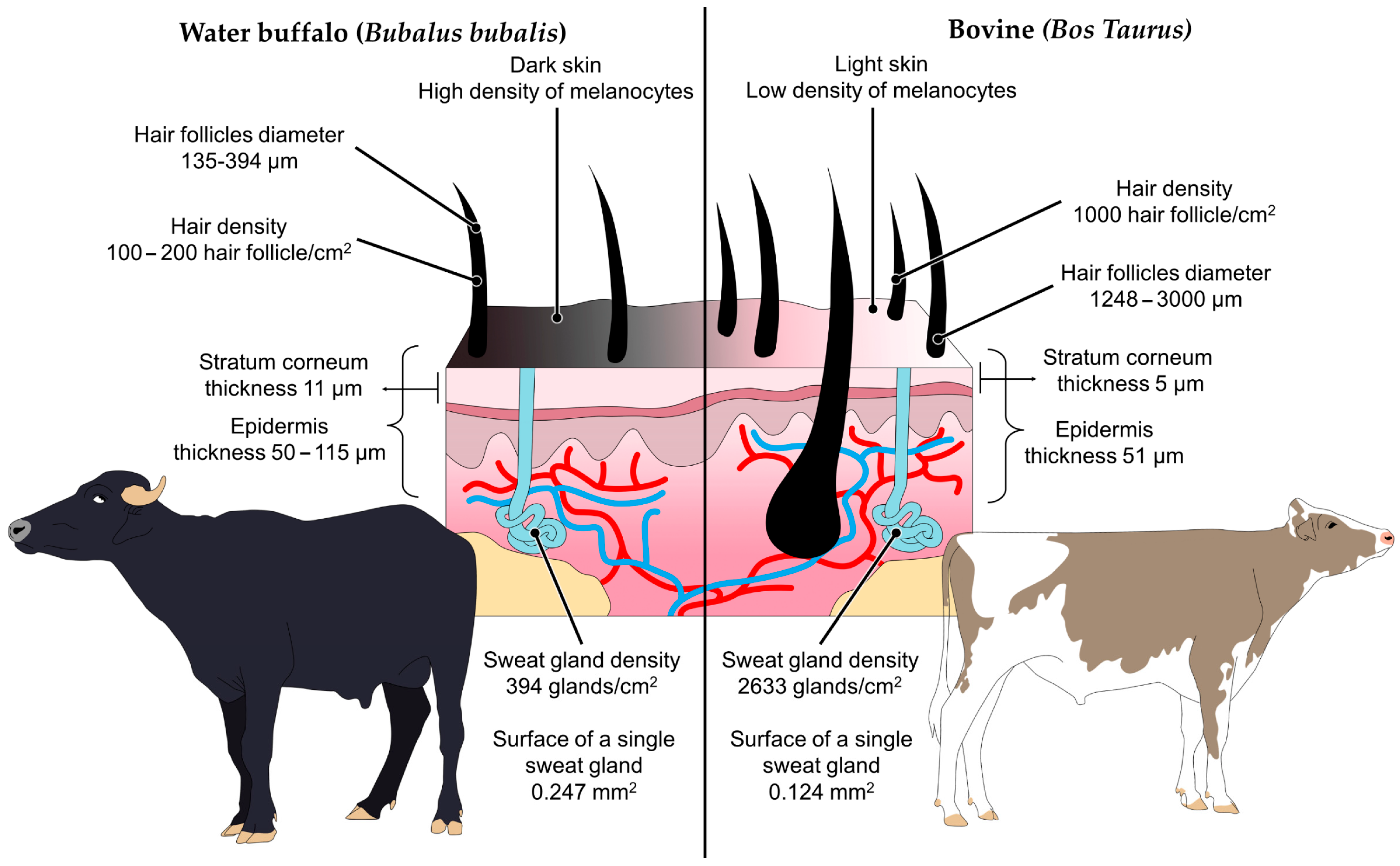This image, likely extracted from a magazine, is a detailed diagram comparing the skin and hair follicles of a water buffalo and a bovine, set against a white background. It is divided by a thin black line running vertically down the middle.

On the left side, there is an image of a black water buffalo, labeled at the top in black text as "Water Buffalo" with its scientific name, "Bubalus bubalis," in parentheses. Below this, a cross-sectional diagram of the water buffalo's skin reveals pink epidermis layered with red and blue capillaries, variously sized light blue sweat glands, and black hair follicles. The hair follicle diameter and density, stratum corneum thickness (11 micrometers), and epidermis thickness (50 to 115 micrometers) are precisely measured and labeled in corresponding black text.

To the right side of the dividing line, there is an image of a brown and white domesticated cow, labeled in black text as "Bovine" with its scientific name, "Bos taurus," in parentheses. Immediately below, a similar cross-sectional diagram depicts the cow's skin, highlighting a lower density of melanocytes, higher hair follicle diameter compared to the water buffalo, and hair density calculated at 1000 hair follicles per square centimeter. The epidermis features red and blue capillaries and smaller sweat glands, which are more densely packed compared to those of the water buffalo. Specific measurements for the stratum corneum and epidermis are also provided.

Overall, the image meticulously contrasts the anatomical differences in skin structure and hair types between the water buffalo and bovine, providing clear, labeled diagrams to illustrate these variations.